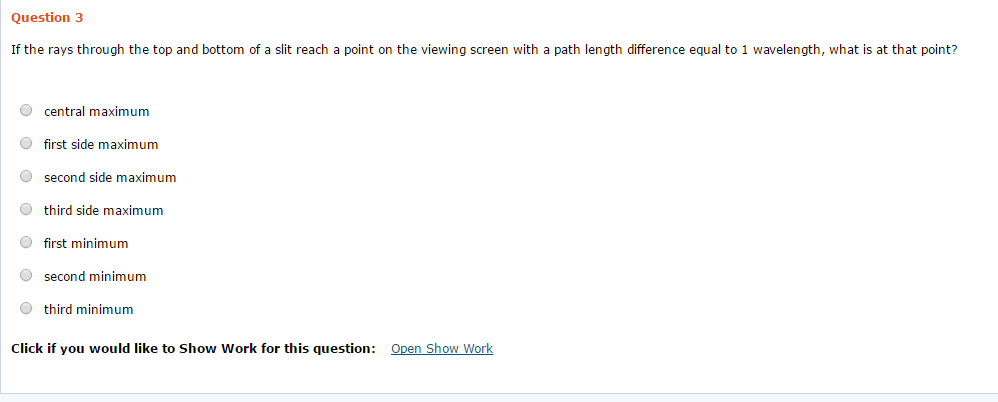A horizontal image prominently features a white background, likely emanating a faint off-white hue from a computer screen. Along the left edge, a very thin black line runs vertically, transitioning into a horizontal black line along the bottom. Below this horizontal line is a gray strip, adding a subtle contrast. The top and right sides of the image remain unembellished, creating a clean border.

In the upper left corner, the text "Question 3" is clearly displayed in orange. Directly beneath this, black text poses a question: "If the ray is through the top and bottom of a slit, reaching a point on the viewing screen with a path length difference equal to one wavelength, what is it at that point?" A series of multiple-choice options follows, each accompanied by clickable circles: central maximum, first side maximum, second side maximum, third side maximum, first minimum, second minimum, third minimum.

At the bottom, bold black text invites interaction: "Click if you would like to show your work for this question." Beneath this instruction, a clickable, underlined option "Open Show Work" appears in blue.